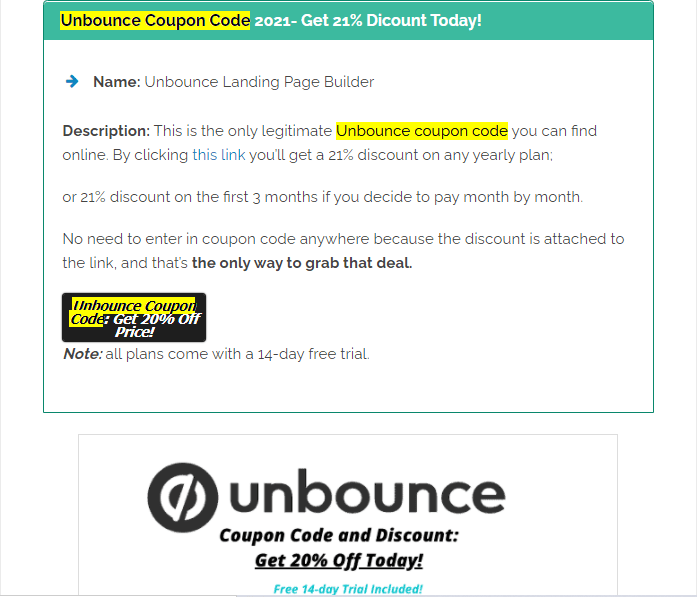This image is a green and white screenshot of an advertisement featured on a web page. At the top, a rectangular yellow-highlighted box displays the text "Unbounce Coupon Code." Below it, the message reads "2021 Dash," followed by "Get 21% discount today" and "discount today" with an arrow pointing towards the "Unbounce Landing Page Builder" name.

The ad's description emphasizes that this is the only legitimate "Unbounce Coupon Code" available online, highlighted in yellow. It mentions that by clicking the provided hyperlink, users can secure a 21% discount on any yearly plan or on the first three months if opting for monthly payments. The discount is automatically applied through the link, eliminating the need for manual code entry.

Placed within a black rectangular box and highlighted in yellow, the "Unbounce Coupon Code" is prominently presented again, stating "Get 20% off price." There’s an additional note indicating that all plans come with a 14-day free trial.

At the bottom-center of the image, there is a black circle logo featuring a white circle slash design. The ad reiterates the offer: "Unbounce is the brand name, coupon code and discount. Get 20% off today. Free 14 day trial included."